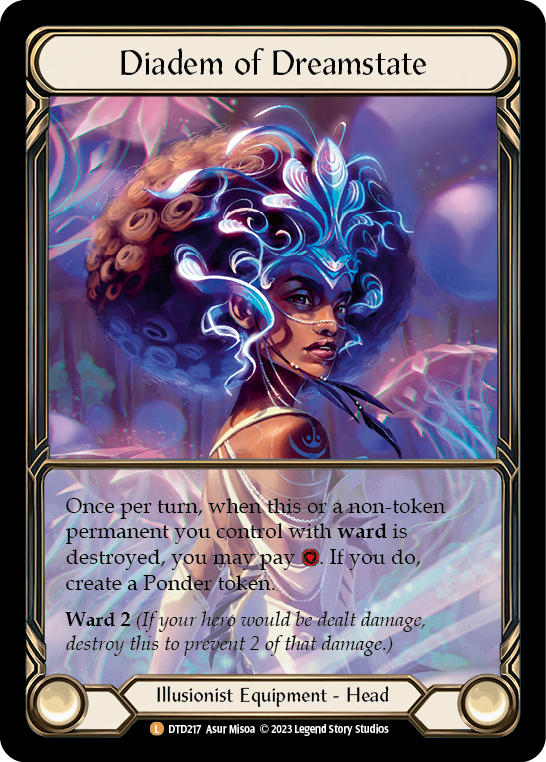The image is a digital screenshot of a trading card featuring an African American woman with a perfectly round, large afro, adorned with a blue, elaborate headdress that extends over her forehead and into her hair. She is depicted wearing a white gown, and the sci-fi themed background behind her consists of hues of purple, blue, and pink, featuring several planets and a mysterious forest. The card has a black border with gold accents and two round yellow knobs positioned at the bottom left and right. At the top of the card on a beige background with black text, it reads "D. Adam of Dream State." Below the illustration, instructions in black text state: "Once per turn, when this or a non-token permanent you control with Ward is destroyed, you may pay [red symbol]. If you do, create a Ponder Token. If your hero would be dealt damage, destroy this to prevent two of that damage. Illusionist Equipment Head." The overall design and text suggest that the card is part of a strategic game set.